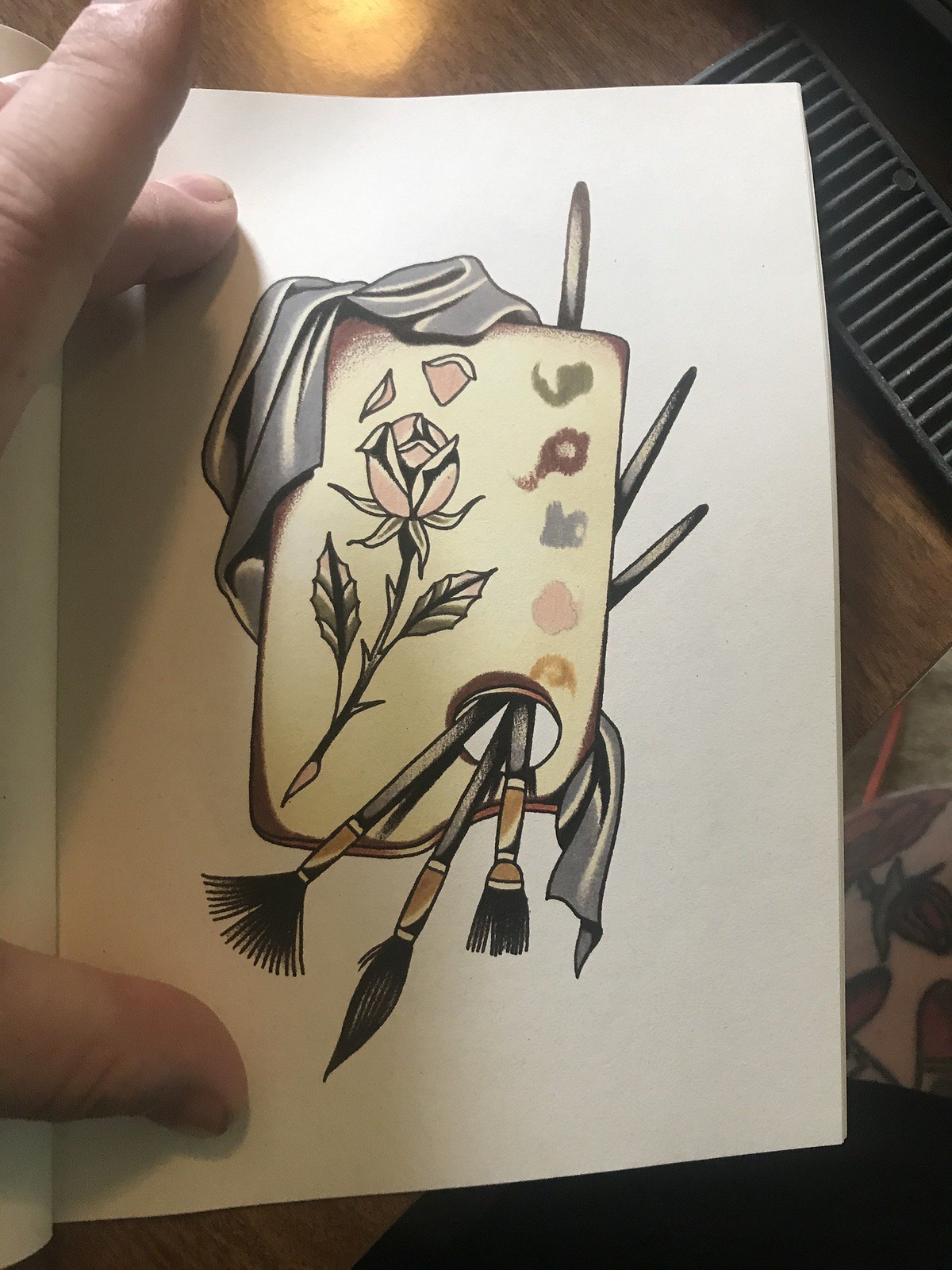The image shows a detailed and precise marker drawing on white paper, seemingly within a book held open by a person's left hand. The hand, whose thumb and middle finger pin down the page while the index finger points out, creates a shadow on the paper. The drawing resembles an artist's palette, a rectangular shape with the bottom right corner cut out, and a hole where a thumb would normally go, but instead, several paintbrushes of varying sizes protrude through. To the right of the palette are vibrant patches of color—green, red, blue, pink, and orange—suggesting paint pools. To the left, a delicately drawn flower with pink petals and pale green leaves stands out, with some petals appearing detached. Additionally, a gray cloth or towel is wrapped around the palette from the top left corner, trailing out to the bottom right. The scenario captures the essence of a creative space, possibly symbolizing an artist's logo or signature work.